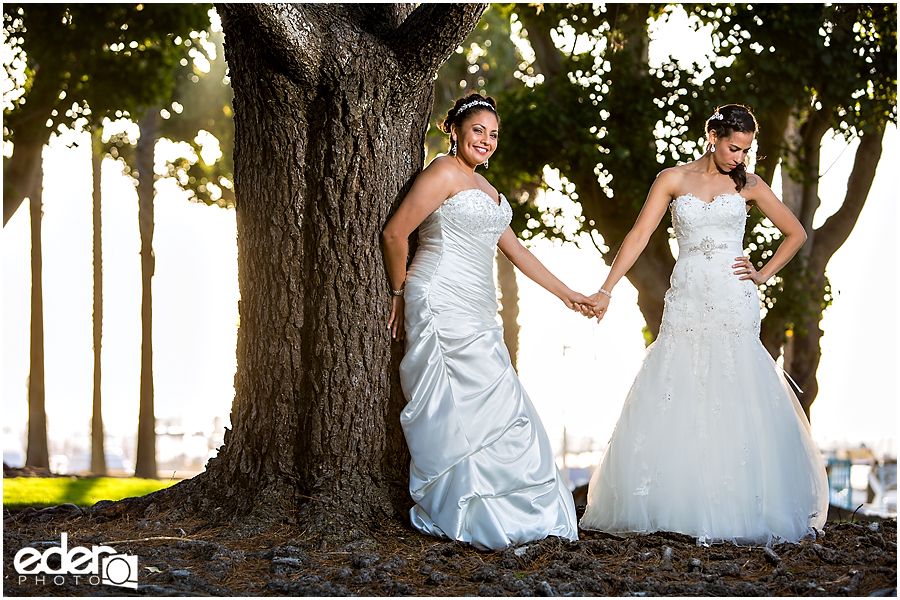This photograph captures a serene and intimate moment between two brides in magnificent white wedding dresses, set against a lush, green park backdrop with a hint of an urban setting beyond the tree line. The bride on the left, adorned in a satin gown with a lace top and a tiara, leans gracefully against a sturdy tree trunk situated slightly left of center. Her radiant smile beams at the camera as she tenderly holds hands with her partner. The other bride, dressed in a mermaid-style lace and tulle gown, stands confidently with her left hand resting on her hip, while her gaze thoughtfully drops downward. Both women have their hair elegantly up and wear matching white bracelets, symbolizing their unity. The ground is covered in moss, suggesting a tranquil ambiance under the sunny sky. In the lower left-hand corner, the photographer's signature and a camera icon read "Eden Photo," marking the artistry behind this beautiful capture.